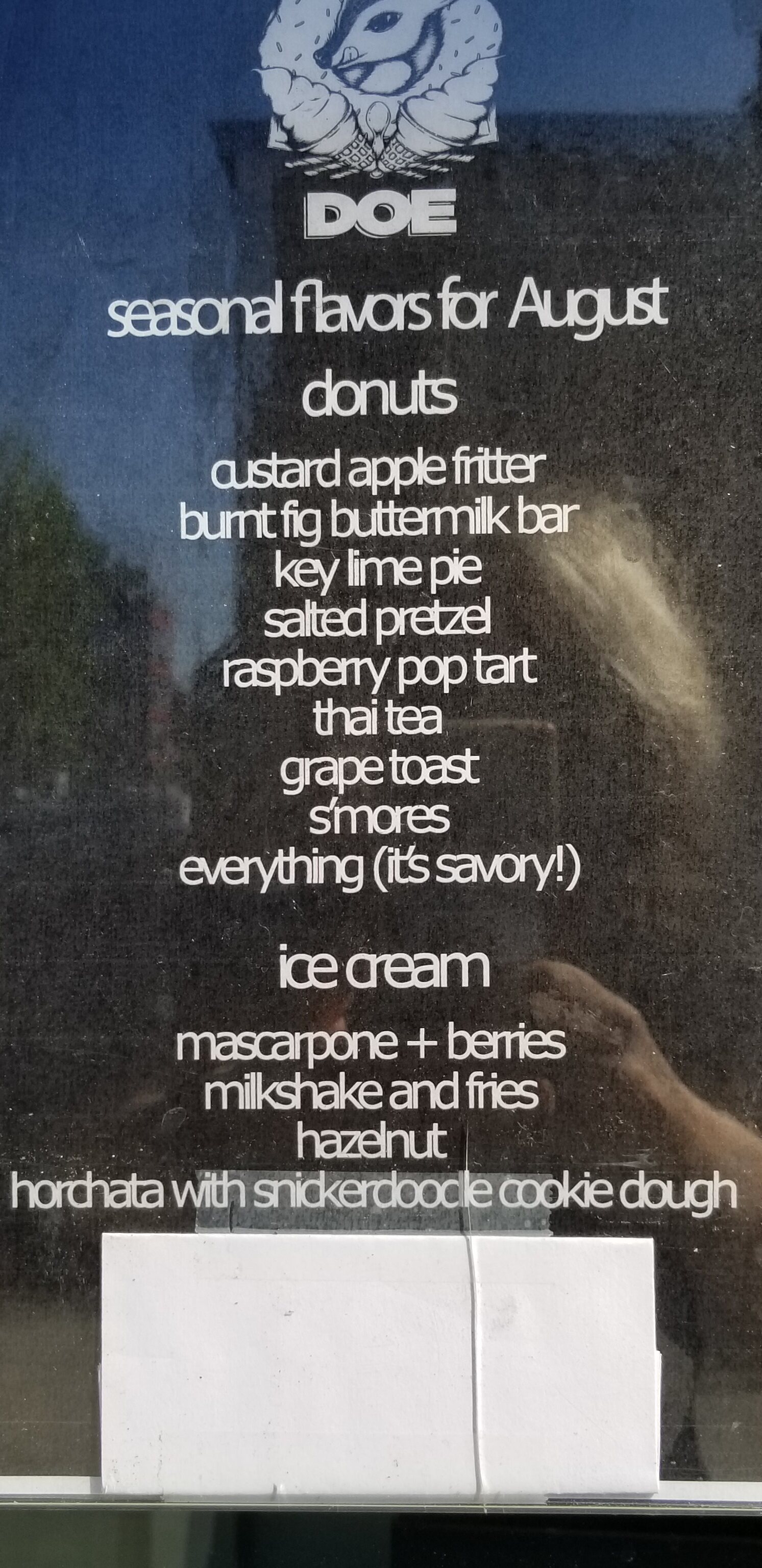A meticulously detailed photograph captures a restaurant's glass menu, intricately etched and filled with the names of delectable seasonal flavors for August. Prominently featured at the top of the menu is the restaurant's logo: a charming emblem depicting a small deer playfully licking its muzzle as it peeks out from a decorative wreath. Adjacent to this, two ice cream cones are artfully arranged to resemble butterfly wings, complete with a spoon forming their central axis. 

In the foreground, a woman is partially visible, holding a sleek silver cell phone in her left hand—her wedding ring glints faintly, suggesting she is married. Her age remains indeterminate, potentially young or perhaps older, adding an air of mystery. She has short, pale hair that could either be white-blonde or purely white.

The focal point, however, is the tantalizing array of dessert offerings from a place named "Doe." The menu lists a delightful range of seasonal flavors: 
- Donuts: Custard Apple Fritter, Burnt Fig Buttermilk Bar, Key Lime Pie
- Salted Pretzel, Raspberry Pop Tart, Thai Tea, Grape Toast
- S'mores Everything (noting in parentheses that it’s savory)

Additionally, their ice cream section boasts flavors like:
- Mascarpone and Berries
- Milkshake and Fries
- Hazelnut
- Horchata with Snickerdoodle Cookie Dough

This woman has captured a mouth-watering snapshot of Doe's seasonal menu, inviting viewers to savor the rich array of flavors through the lens of her camera.